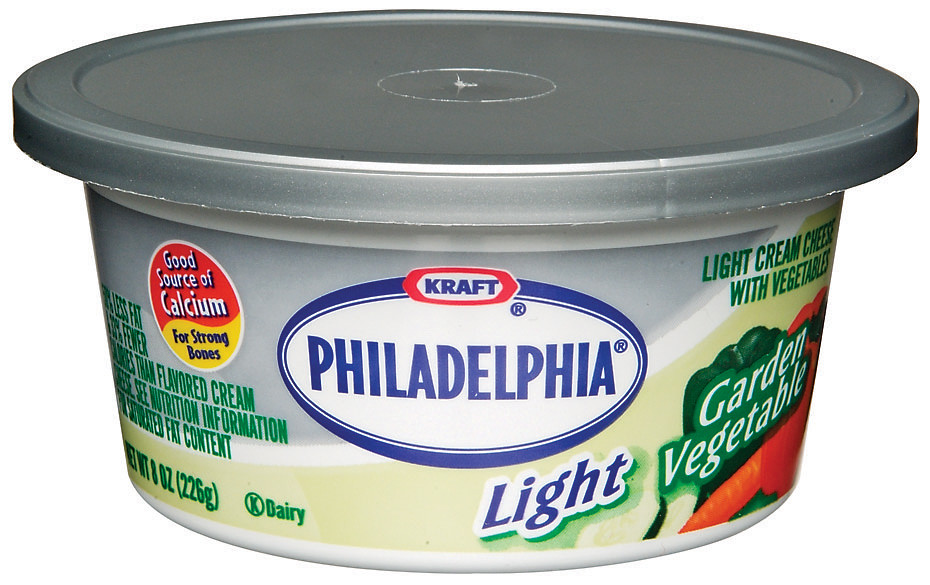This close-up image features a circular 8-ounce container of Philadelphia Garden Vegetable Light Cream Cheese with Vegetables, prominently branded by Kraft. The tub is made of plastic with a light gray, round lid. The label showcases the Philadelphia logo in blue capital letters against a white background, with a blue outline and a red oval framing the Kraft logo. The container's detailed design includes pictures of vibrant orange carrots and green bell peppers indicative of the garden vegetable flavor. To the right-hand side of the container, "garden vegetable" is noted, along with the product's light cream cheese designation. A smaller red and yellow circular logo on the left side emphasizes the product's nutritional benefits, stating it is a good source of calcium for strong bones. Additional information highlights that the product has less fat and fewer calories than other flavored creams, encouraging consumers to check the nutritional details. The package, also marked as an 8-ounce (226-gram) dairy product, features descriptive green text about its nutritional content and fat percentage. The swirling white band and light tan color beneath the label enhance its visual appeal, making it a familiar and recognizable item on the shelf.